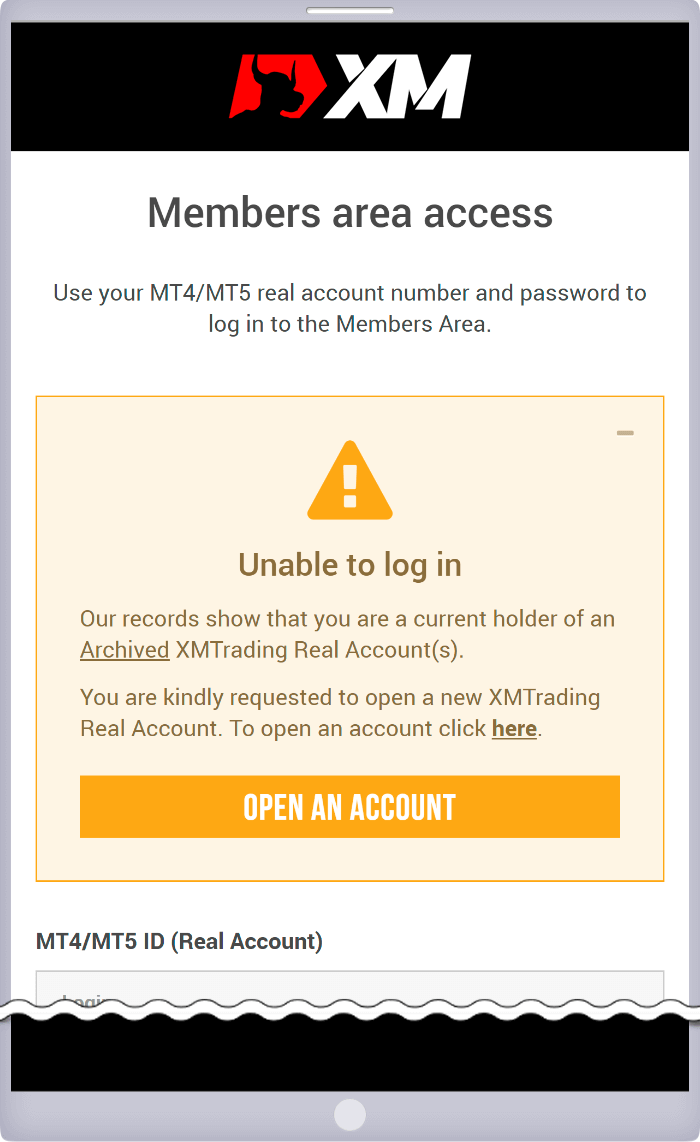**Detailed Caption:**

The screenshot displays a "Member Access Only" area with a clean and structured layout. At the top of the screen, a prominent black bar spans the width of the page. Below this, a red solid arrow points towards the left, accompanied by an outline resembling a bowl. Inside the bowl-like outline, the letters "XM" are prominently displayed in white font.

Beneath this section is a white area which contains black text that reads, "Member Access. Use your MT4/MT5 real account number and password to log into the member area." 

Directly below the instructions, an orange box is featured. This box includes an orange triangle with a solid fill and an exclamation mark inside, surrounded by a light orange background. The accompanying text states, "Unable to log in. This indicates that you are a current account holder. This is the new XTM trading real account. Open an account over here."

At the very bottom of the screenshot, an orange bar is displayed with white text that says, "Open an account." Below this bar is a decorative squiggly line followed by a smaller black bar. On the bottom-right side, there is a tiny circular dot.

This organized and polished layout ensures users have clear instructions and navigational options for accessing or creating their accounts.